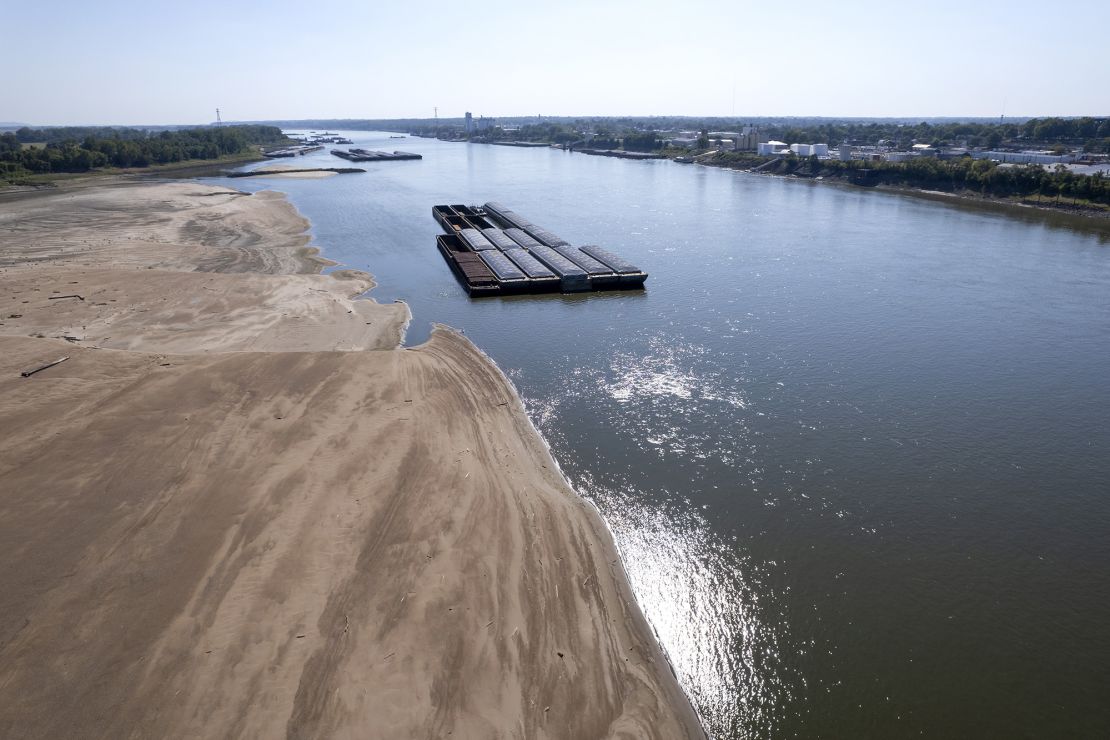The image depicts a vast river, with a sprawling earthy brown shoreline on the left side, extending about three-quarters up the picture. The water, a mix of murky and blue hues, features several flat, rectangular containers of varying colors, brown and gray, some floating near the silty shore and others scattered further out. The right side of the image reveals a picturesque town or city, enveloped by lush green trees and a few tall buildings framed by a clear blue sky. In the background, several wind turbines are quietly nestled among the trees, adding a serene yet industrious element to the landscape. The entire scene is bathed in natural, earthy tones, enhancing its tranquil and expansive beauty.